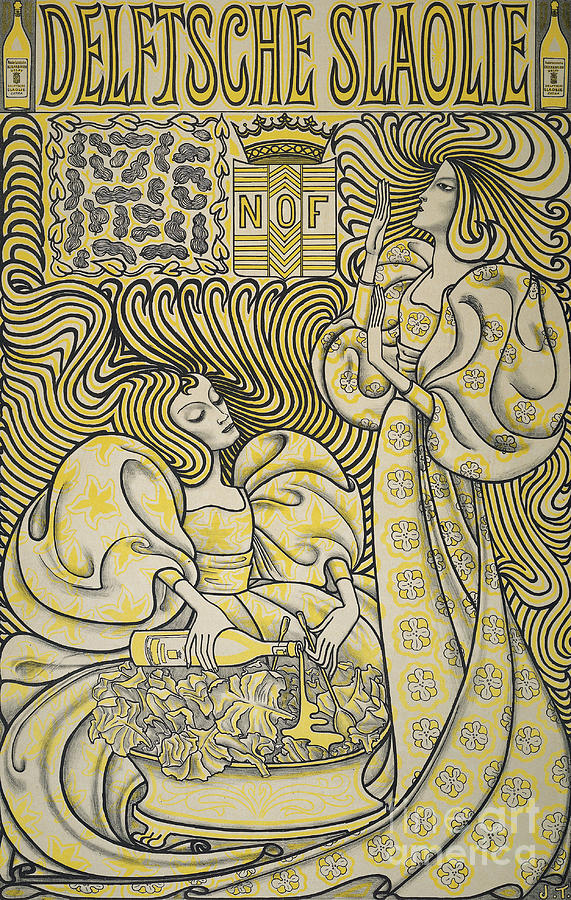This richly detailed, stylized illustration, possibly a woodcut or screen print, employs a limited color palette of navy, blue, tan, yellow, black, gray, and white. The tan color of the paper gives it a textured, almost vintage feel. The scene centers on two elegantly elongated women adorned in flowy dresses with billowing, puffed sleeves that taper at the wrists. The standing woman on the right extends her hands in front of her, contributing to the swirling motion that permeates the artwork. Her intricate hair, like that of her seated counterpart, forms dramatic, swooping lines that dominate the background.

The seated woman on the left is intently mixing a salad in an impressively large, claw-footed bowl. She carefully pours a liquid, potentially a balsamic vinaigrette, from a tall, narrow bottle while holding a mixing spoon in her other hand. This bottle resembles the style of an alcohol or wine bottle, adding to the elegance of the scene.

Art Deco lettering at the top of the image spells out "DELFTSCHE SLAOLIE," accompanied by a detailed crest featuring the letters "N-O-F" set against yellow and white stripes and crowned with an intricate design. Small bottles flanking the text on both sides enhance the visual balance. A watermark in the lower right corner subtly reads "Art America," grounding the piece in its artistic context.